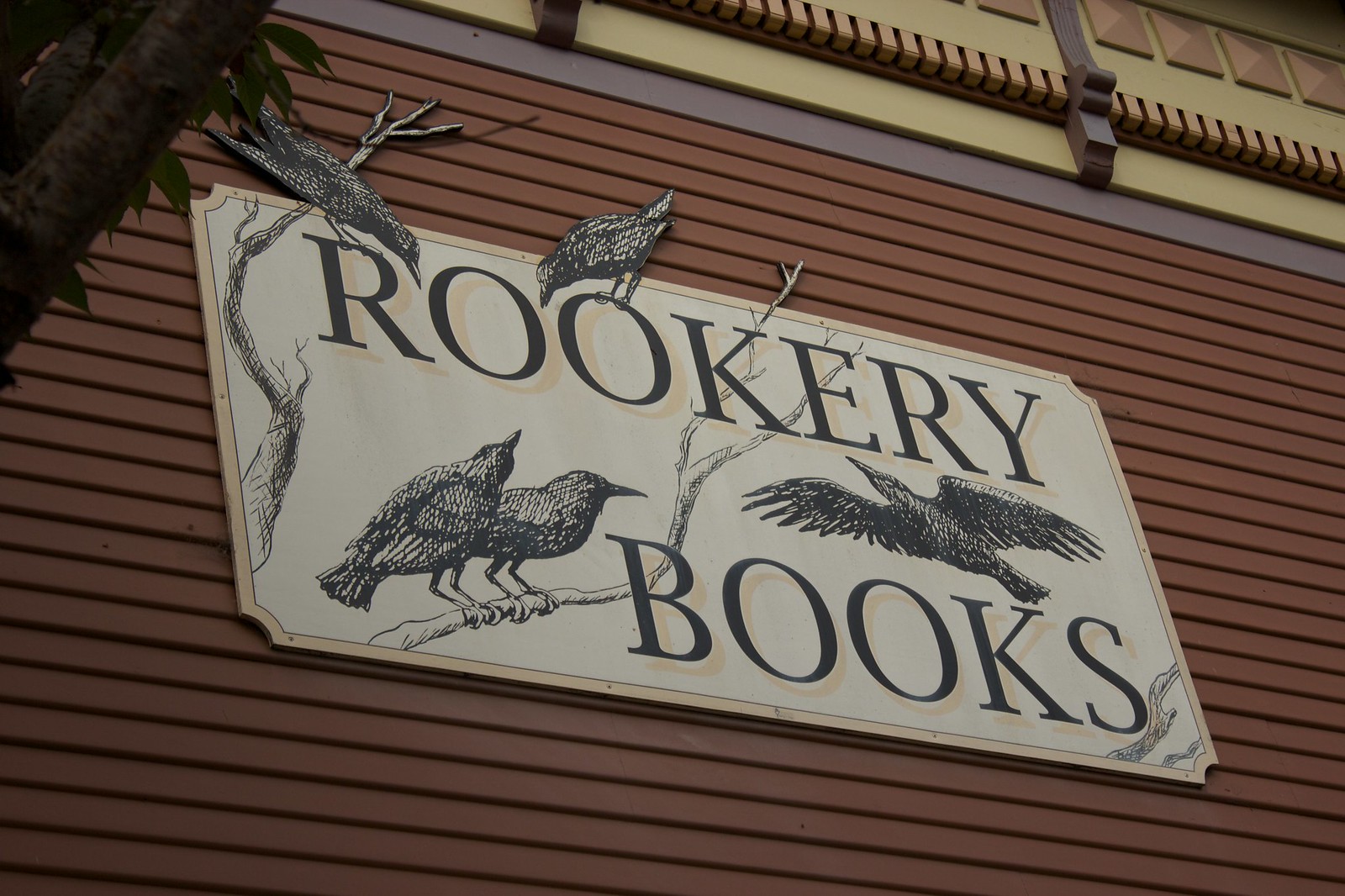The image depicts the side of a building with planked, reddish-brown siding. Affixed to the center of this wall is a large, rectangular, cream-colored sign with black lettering that reads "Rookery Books." The sign features illustrations of crows or rooks perched on branches, with two birds sitting on branches between the words and one crow flying above the word "Books." Additionally, there are two crows perched on the top of the sign, specifically on the letters "R" and "O" of "Rookery," and these birds project out slightly beyond the sign's border. A tree with a brown trunk extends diagonally from the upper left corner of the image, with branches slanting into the frame. Above the reddish siding, a thin strip of purple is visible, followed by a section of yellow molding adorned with evenly spaced, small, square projections that align along the building's facade.